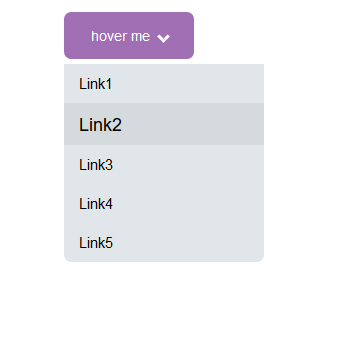The image depicts a vertical, unbounded screenshot of a drop-down menu on a white background. At the top of the image is a purple rectangular button with curved edges, featuring the white text "hover me" in all lowercase, accompanied by a downward-pointing white arrow. When users interact with this button, a drop-down menu appears below it. The menu consists of five links listed vertically: "Link 1," "Link 2," "Link 3," "Link 4," and "Link 5." Each link has black text on a grey background, with "Link 2" slightly highlighted in a darker grey. This interface element suggests a dynamic menu that appears upon hovering and allows users to interact with the listed links.